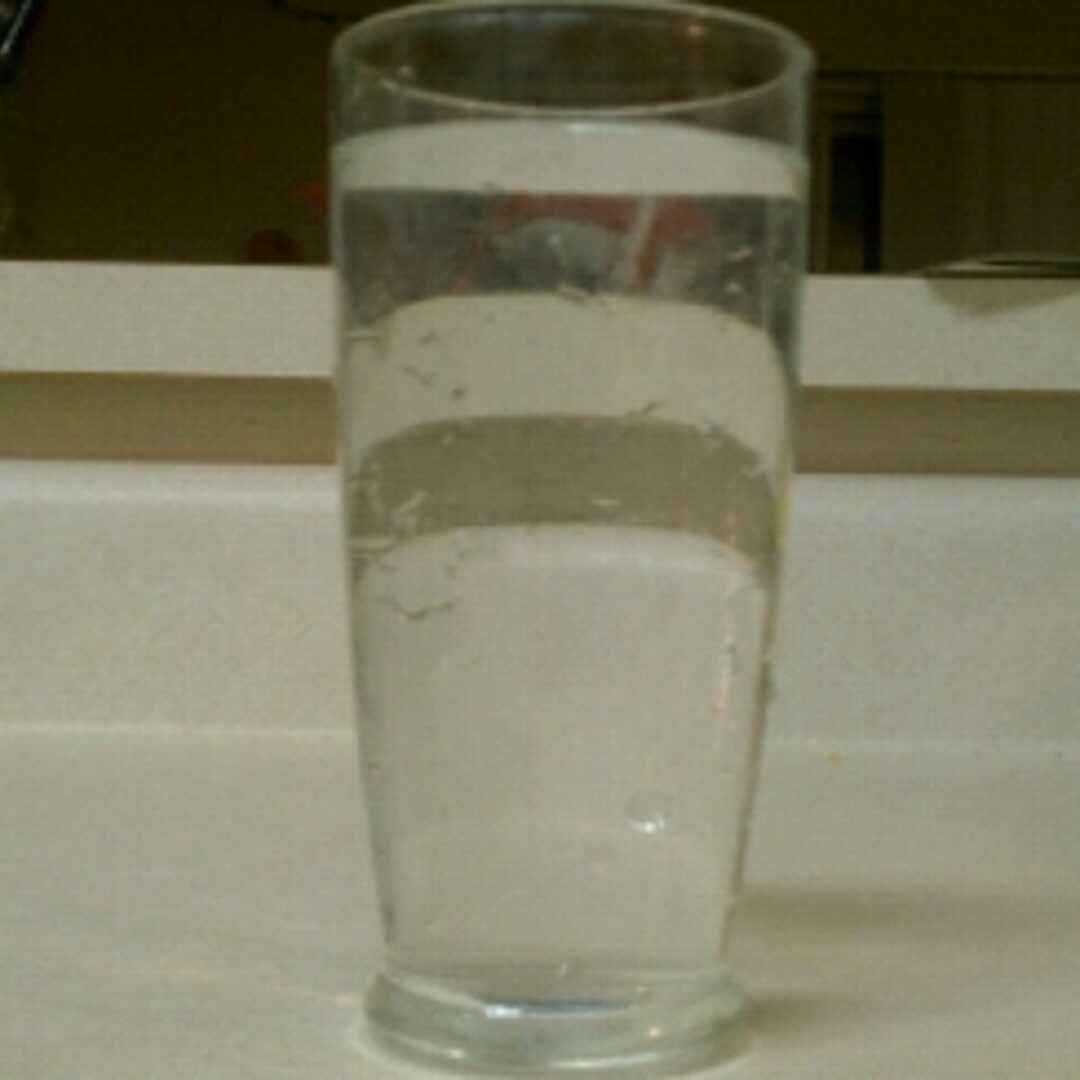In the foreground of the image, a large, clear glass filled nearly to the brim with cold water is placed on a pristine white countertop. The outside of the glass is wet with condensation, indicating it might have contained ice or been recently washed. The main focus of the image, the glass, captures the viewer’s attention due to the close-up shot that emphasizes its coldness and the water droplets clinging to its surface. Through the glass, the silhouette of the photographer can be vaguely seen, hinting at someone wearing a red shirt. The countertop stretches across the picture, featuring a sleek design with a tan wood trim. Despite the close focus on the glass, a magazine or book is faintly visible on the counter, along with a suggestion of window curtains, possibly light tan in color, in the dimly lit background. The overall noise and high ISO characteristics suggest that the image was digitally zoomed in, adding to its grainy texture. The setting appears to be a kitchen or a living room area with a floating island bar, though specific background details remain indistinct.